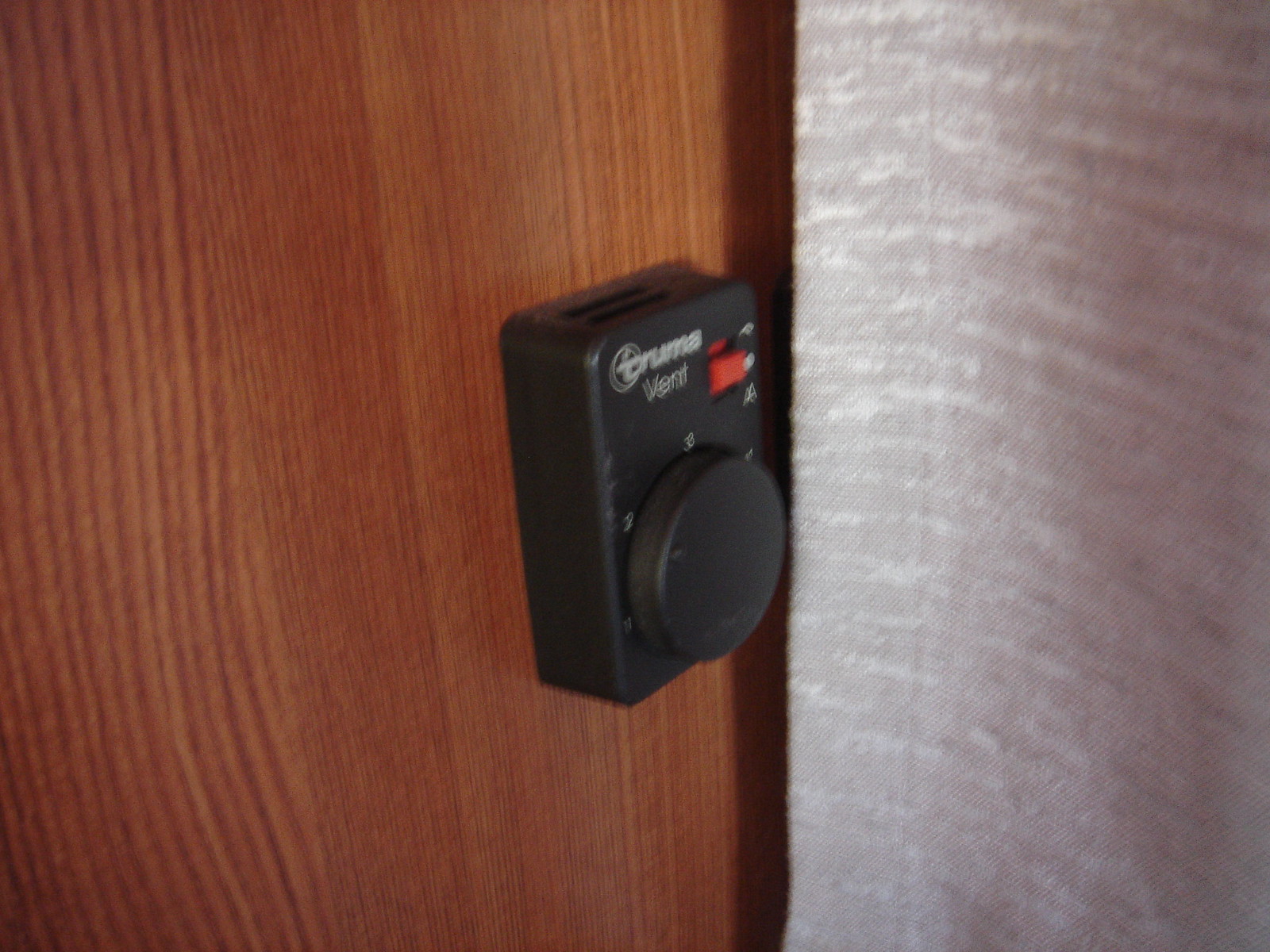The image depicts a black thermostat mounted on a textured wooden wall. The wall features a rich walnut hue with varying light, dark, and orangish-brown grains arranged in a grooved pattern. The thermostat, marked with white lettering, includes a knob labeled from one to four and a red on/off switch situated on the lower right. To the right of the thermostat hangs a white curtain, which has subtle, almost shiny, light white flecks woven into the fabric.